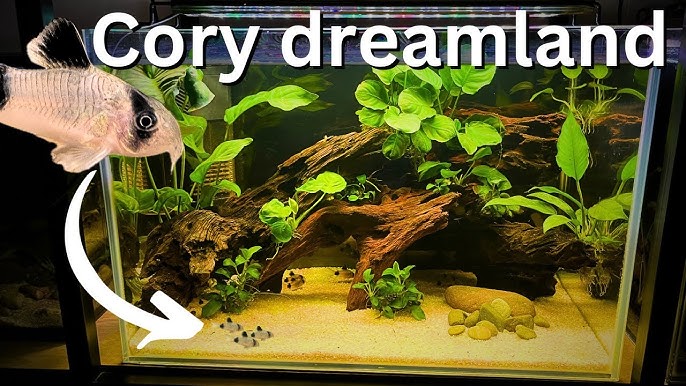This is a detailed photograph of a large glass aquarium labeled "Kori Dreamland" in bold white letters at the top. The tank features an abundance of wooden branches, logs, and lush greenery, creating a vibrant and natural aquatic environment. The bottom is covered with white gravel and some rocks, providing a base for the setting.

Within the aquarium, there are six fish—three at the bottom are highlighted by an arrow in the image. These fish are white with distinctive black banding on their fins, tails, and around their eyes. In the top left portion of the photograph, there is an inset image of the same fish species, further emphasizing their appearance. These fish, identified as Kori, are the exclusive inhabitants of the tank. The background outside the tank is indistinct, possibly showing parts of furniture like stool legs. This aquarium is vividly portrayed as an ideal habitat for the Kori fish, showcasing both their unique appearance and their serene environment.